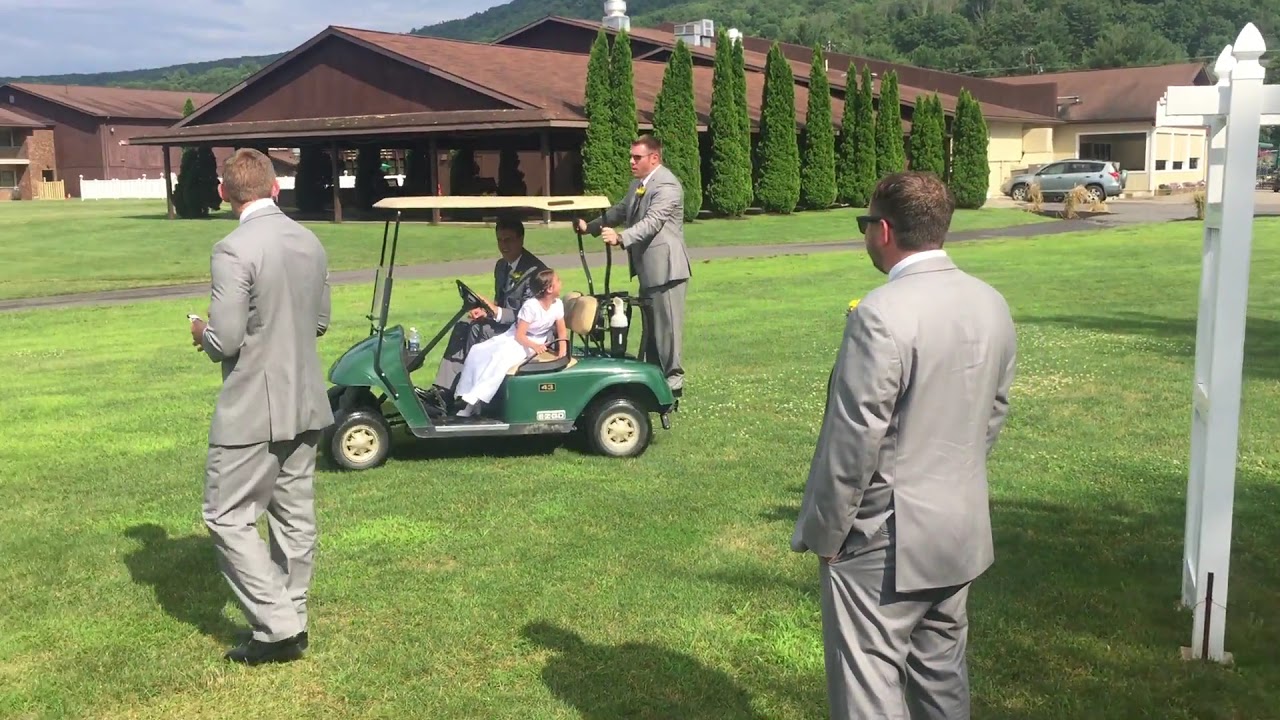This photograph captures a wedding scene set on a lush, green golf course, characterized by a group of men in matching light gray suits accented with yellow flowers on their lapels. Central to the image is a dark green golf cart, positioned facing the left, with a white man in the passenger seat and a young Caucasian girl in a white dress sitting beside him, presumably driving. On the back of the golf cart, a third man, also in a gray suit and wearing sunglasses, appears to be riding along. Surrounding the cart are two more white men in identical gray suits, their backs to the camera.

The background of the image features a dark brown wooden building with brown roof tiles, hinting it might be the event space. On the right side of the frame, partly cut off, is a white ceremonial arch, suggesting the wedding ceremony may have taken place nearby. Further details in the backdrop include a silver SUV parked near another extension of the building, which appears to be a bright yellow color, along with a walkway stretching across the scene. Sculpted trees and bushes line the building, adding to the manicured, picturesque setting, while a distant hill and forested area rise towards the top left, completing the serene landscape.